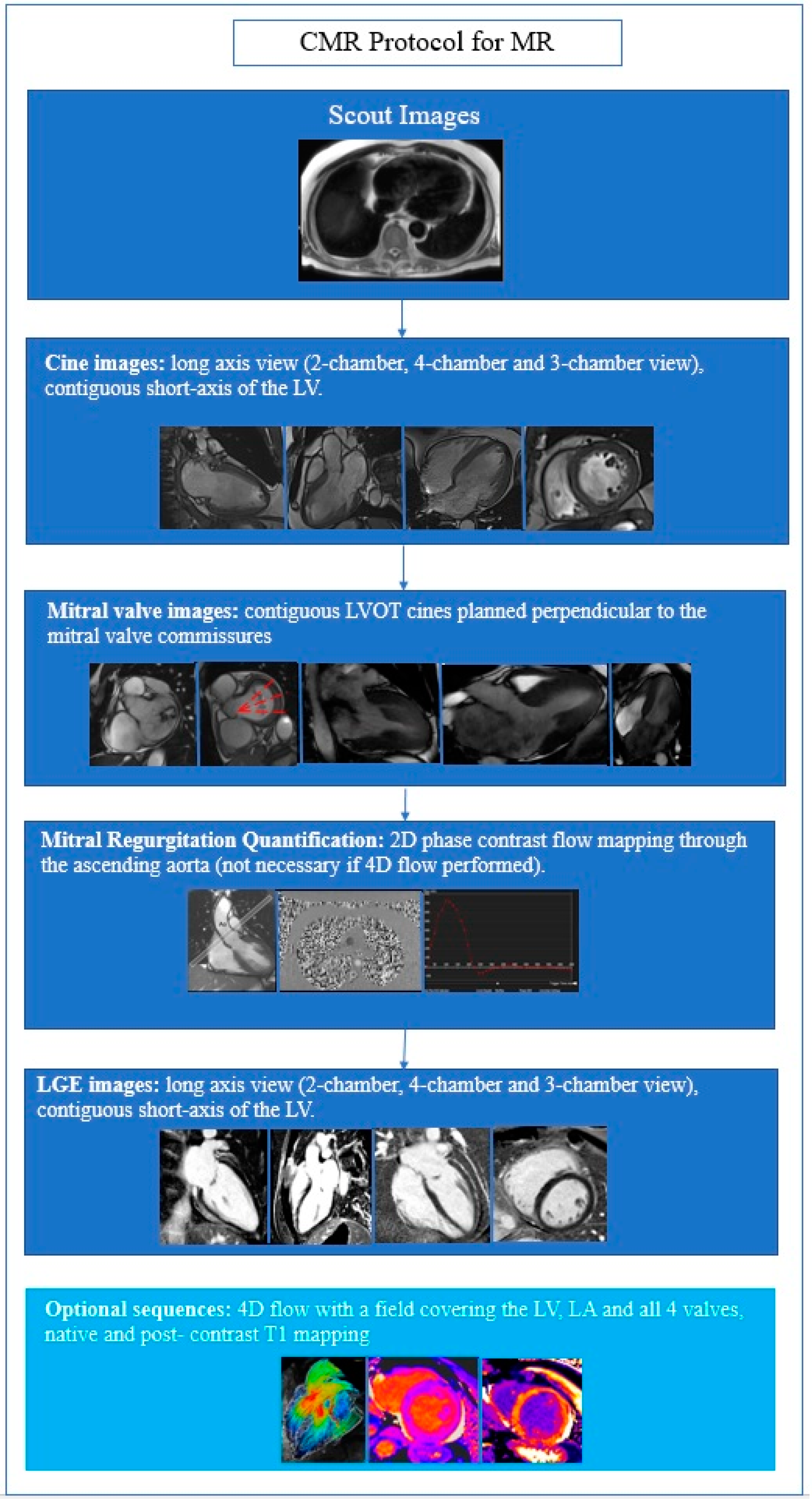The image depicts a medical informational page with a white background, divided into six horizontal blue sections, each containing specific content related to the CMR protocol for MR. At the top, in a box outlined in thin blue, the title "CMR Protocol for MR" is displayed in black letters. The first blue section, labeled "Scout Images" in white text, features a black and white X-ray, possibly of a brain. 

The second section, labeled "Synth Images Long Axis View," includes four black and white images displaying long axis views of the heart, with two-chamber, four-chamber, and three-chamber views, and continuous short axis images of the LV. 

The third section, titled "Mitral Valve Images," provides images of the mitral valve in continuous LVOT signs, planned perpendicular to the mitral valve commissures, and contains five X-ray images. 

Below this, the fourth section labeled "Mitral Regurgitation Quantification" shows three images related to 2D phase contrast flow mapping through the ascending aorta, noting that this step is unnecessary if 4D flow is performed.

The fifth section, titled "LGE Images," includes four X-ray images showing long axis, two-chamber, four-chamber, and three-chamber views, along with continuous short axis images of the LV.

The final section, labeled "Optional Sequences," displays colorful heat map X-ray images of the heart, specifically a 4D flow covering the LVLA and all four valves, along with native to post-contrast T1M mapping, with three such images in a row.